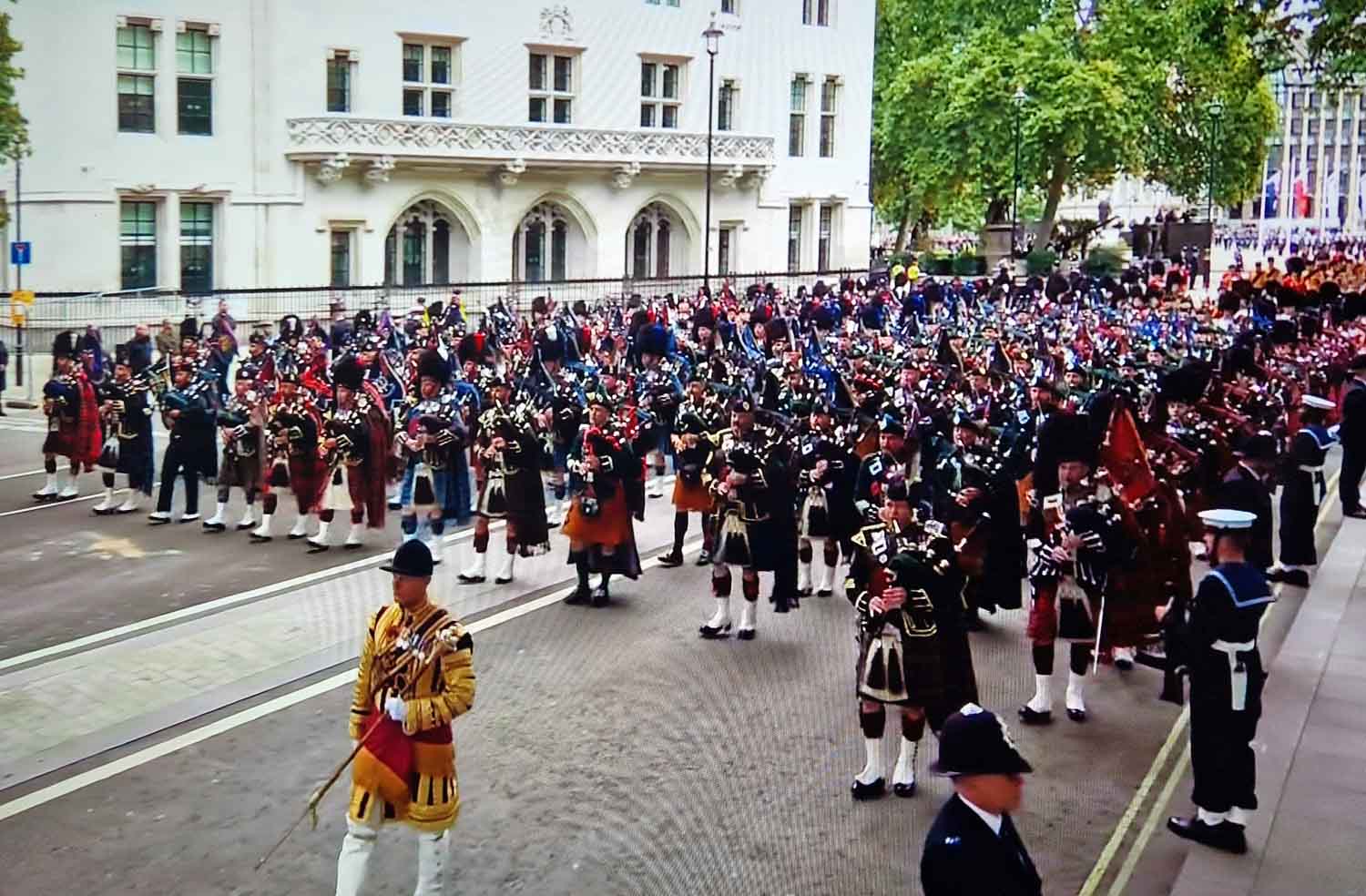Captured in an outdoor, daytime setting, this image appears to be from a parade or ceremonial procession, likely taking place in a street reminiscent of those in Scotland, England, or perhaps even Ireland. Central to the scene is a large Scottish marching band consisting predominantly of men dressed in traditional kilts. Each of them is playing a bagpipe, with uniformity suggesting they are performing in rhythm. The sea of bagpipers stretches back for numerous rows, creating an impressive display of coordinated musicianship.

The focal point of the image is a man dressed in a striking yellow uniform who seems to be directing the band, possibly a drum major or band leader. He holds a large, ornate staff, which he uses to guide or signal the musicians behind him. Surrounding the parade on either side of the street are a mix of onlookers and uniformed personnel—black and white clad sailors and police officers can be seen standing vigilantly, with sailors holding rifles upright.

Despite the street resembling a typical urban setting with buildings in the background, the image itself has a digital screen appearance, complete with visible scan lines, as if it’s a photograph of a television or monitor. This adds an additional layer to the scene, possibly indicating that it depicts footage from Queen Elizabeth II's funeral procession, given the formal and elaborate nature of the march and the mixture of military and civilian presence.